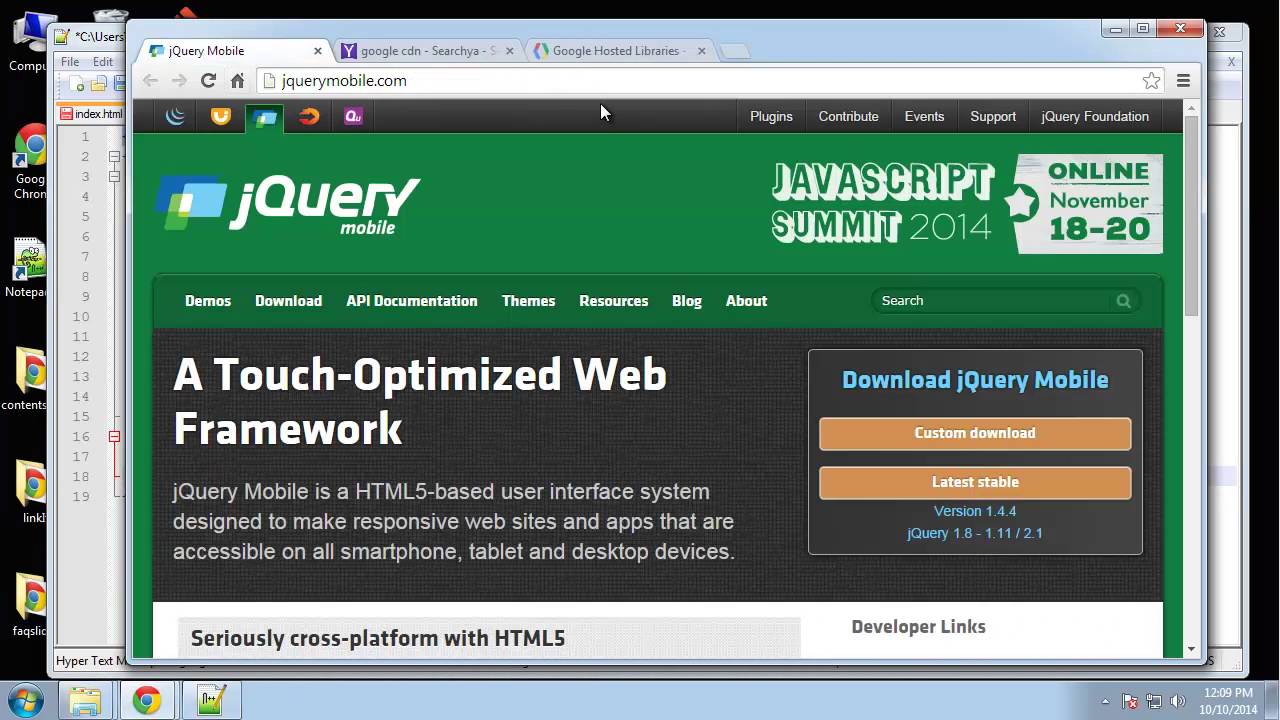Captured on October 10, 2014, at 12:09 PM, this image reveals a snapshot of a computer screen displaying a detailed interface related to jQuery Mobile and its JavaScript Summit 2014 event scheduled for November 18-20. At the top of the screen, a flag is visible, accompanied by text indicating "Bon Alumni." The bottom of the screen features icons of a Microsoft Windows folder, Google Chrome, and a notepad application. The main content showcases the TouchOptimus framework, jQuery Mobile, and various navigation options such as "Demo," "Download," "API Documentation," "Themes," "Resources," "Blog," and "About."

Prominently placed on the right side, there is a call-out to "Download jQuery Mobile," including two orange rectangles that draw attention to the version details: "Version 1.4.4, jQuery 1.8, 1.11 / 2.1." The left side describes jQuery Mobile as an HTML5-based user interface system designed to make responsive websites and apps compatible with all smartphones, tablets, and desktop devices. Below this, developer-related links are listed with a note affirming the timestamp, "This is 10.10.2014."